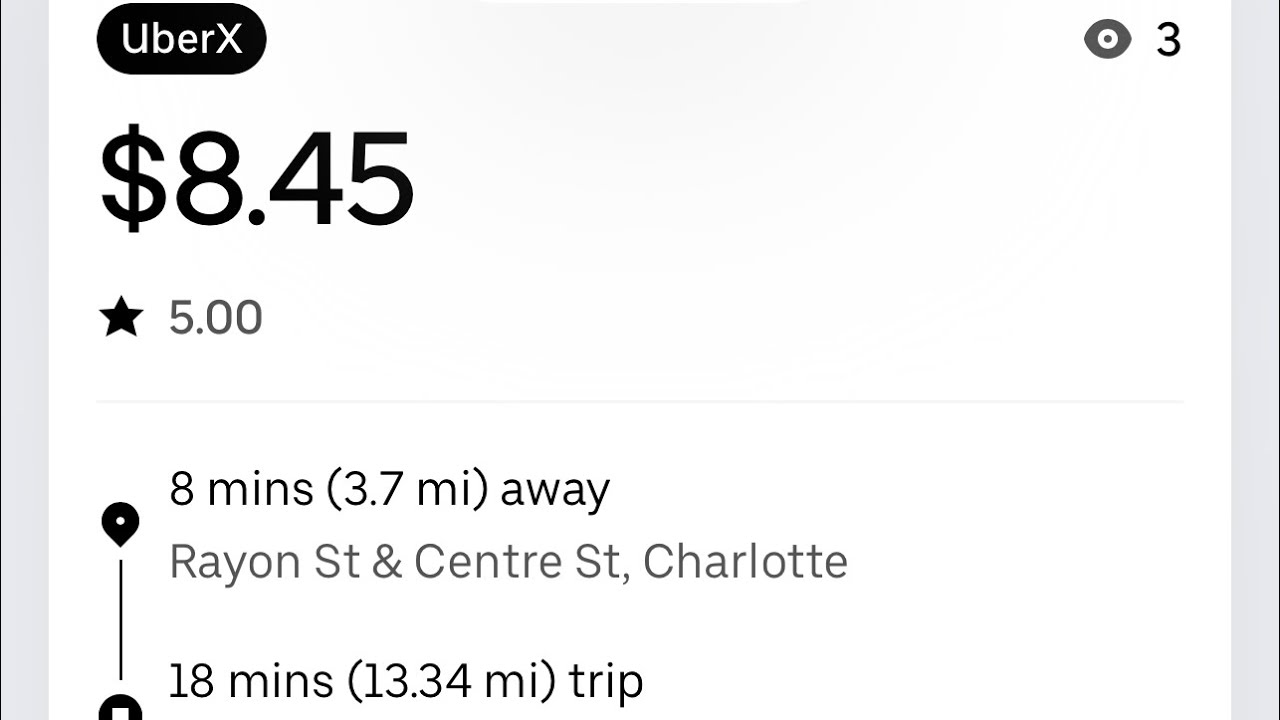"UberX ride estimated at $8.45, rated 5 stars, will arrive in 8 minutes. The destination is 3.7 miles away, near the intersection of Rain Street and Center Street in Charlotte. The total estimated travel time for the 13.34-mile trip is 18 minutes. The image features a white background with black text. There is a dark drawing and a white sketch, with both visuals comprising black and white elements."